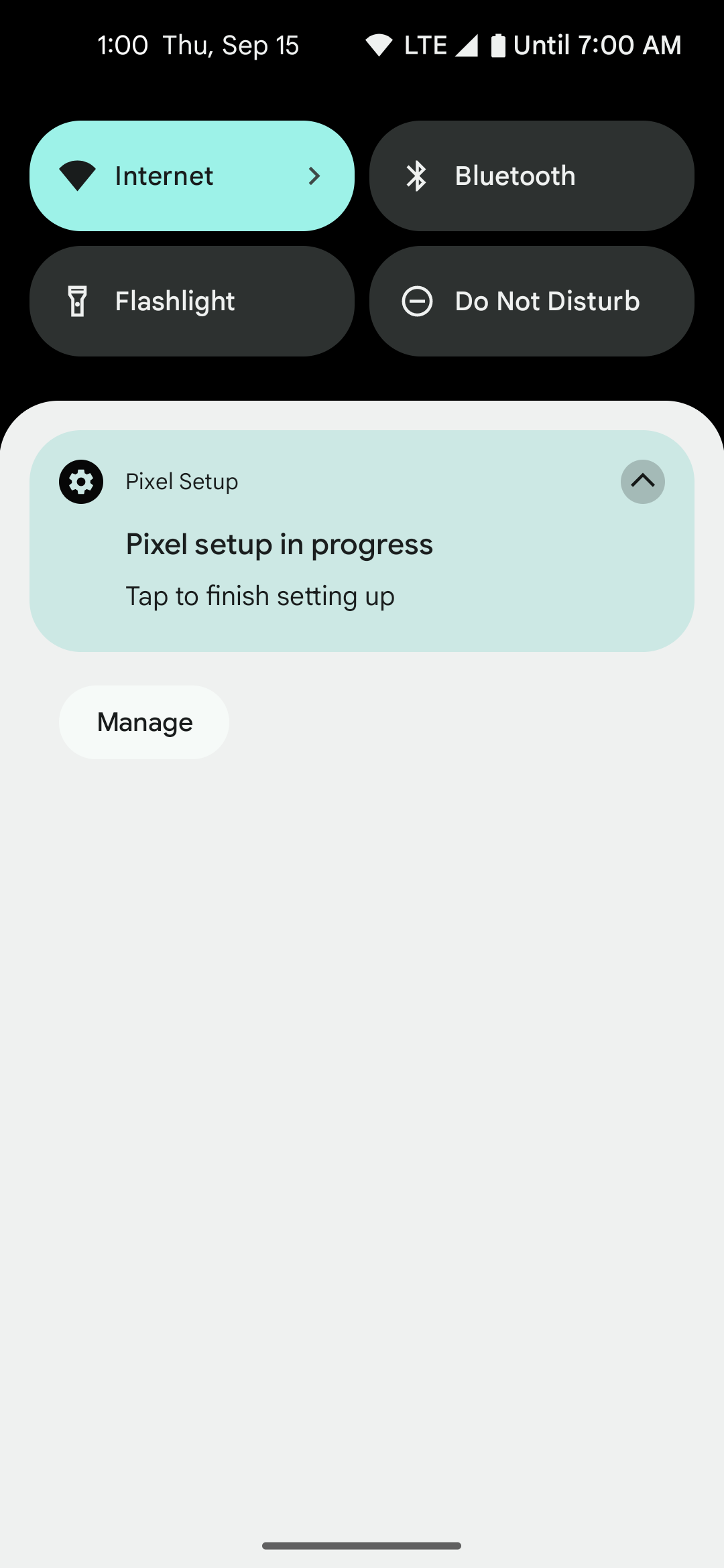The image displays the status bar and setup screen of a mobile device. It is 1 o’clock on Thursday, September 15th. The status bar shows full LTE signal strength and a fully charged battery with an estimated endurance until 7 AM. Icons indicate that internet and Bluetooth are active, while the flashlight and 'Do Not Disturb' mode are not activated.

In the center of the screen, under the heading "Pixel Setup," there is a text indicating that the setup is in progress. It prompts the user with "Time to finish setting up" and provides an option to "Manage." A horizontal line is present at the bottom of this section.

Overall, the image portrays various details related to the device's connectivity and setup process in progress.